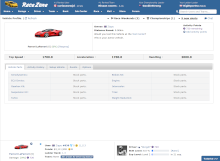The image depicts a section of a car-related website. At the top, there's a prominent banner displaying the text "Race Zone" along with an image of an orange sports car. The main part of the website features a striking red sports car against a clean, white background. Beneath the image of the red car, there are several tabs presumably for more information. Further down, at the bottom of the page, there are additional clickable links designed to navigate various sections of the website or redirect to other external resources. While the specific details are small and somewhat unclear, the overall layout and imagery suggest that the site is dedicated to either showcasing, selling cars, or offering car-related parts and services.